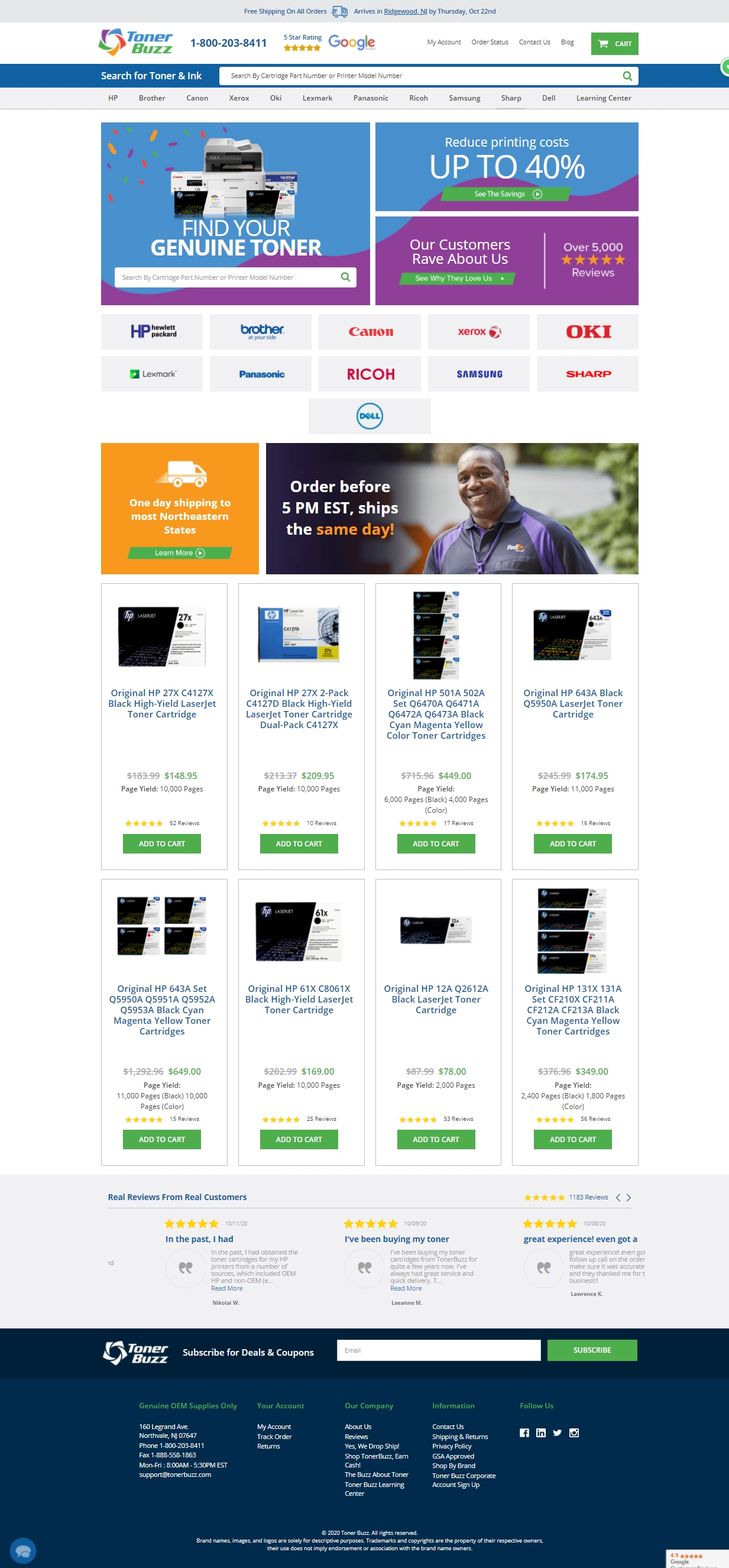This image, captured from a smartphone screen, displays a webpage for Toner Buzz. At the top, it shows a search field indicating the user is looking for information about the company. The page prominently displays Toner Buzz's contact number, 1-800-203-8411, and boasts a five-star rating with five vivid yellow stars next to the multicolored Google logo.

Just below, the navigation bar contains links labeled "My Account," "Order Status," "Contact Us," and "Blog," alongside a green "Cart" button. Further down, there's a search prompt titled "Search for Toner and Ink," with options to search by Cartridge, Part Number, or Prime Mobile Number.

The middle section of the page features an image of various printers along with a header that reads "Find Your Genuine Toner." Below this, there are two rows of products, each containing four items that users can click to add to their cart. Every product listing includes reviews just above the green "Add to Cart" button.